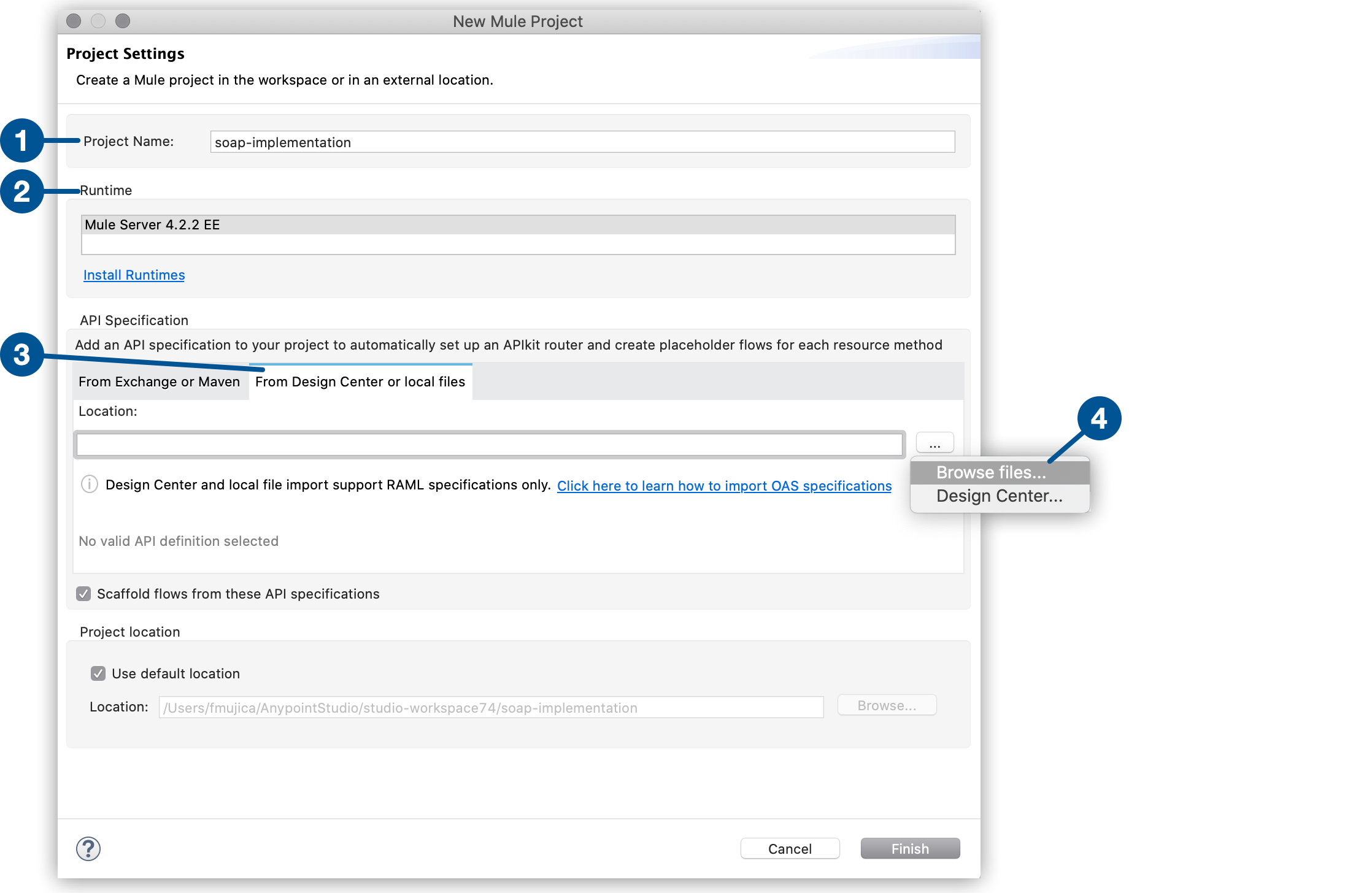This grayscale screenshot captures a Mac application interface, specifically the setup window for creating a new Mule project. The top of the screen features a horizontal gray bar with the title "New Mule Project" centered within it. In the top left corner of the screen, characteristic of Mac applications, are three circles, typically red, yellow, and green, but shown here in grayscale. This distinguishes the platform as macOS, unlike Windows which places similar controls in the top right corner.

In the upper left section of the window, bold text reads "Project Settings," followed by the description "Create a Mule Project in the Workspace or in an External Location." Below this, the interface offers various configuration options including fields labeled "Project Name," "Runtime," and "API Specification," among other settings and checkboxes that allow users to customize their Mule project environment.

At the very bottom of the screen are two prominent action buttons. Positioned in the bottom right corner, there is a white "Cancel" button with black text, and adjacent to it, a dark gray "Finish" button with white text. Additionally, in the bottom left-hand corner, a help icon represented by a question mark inside a black circle is visible, indicating where users can find more information or assistance with the setup process.